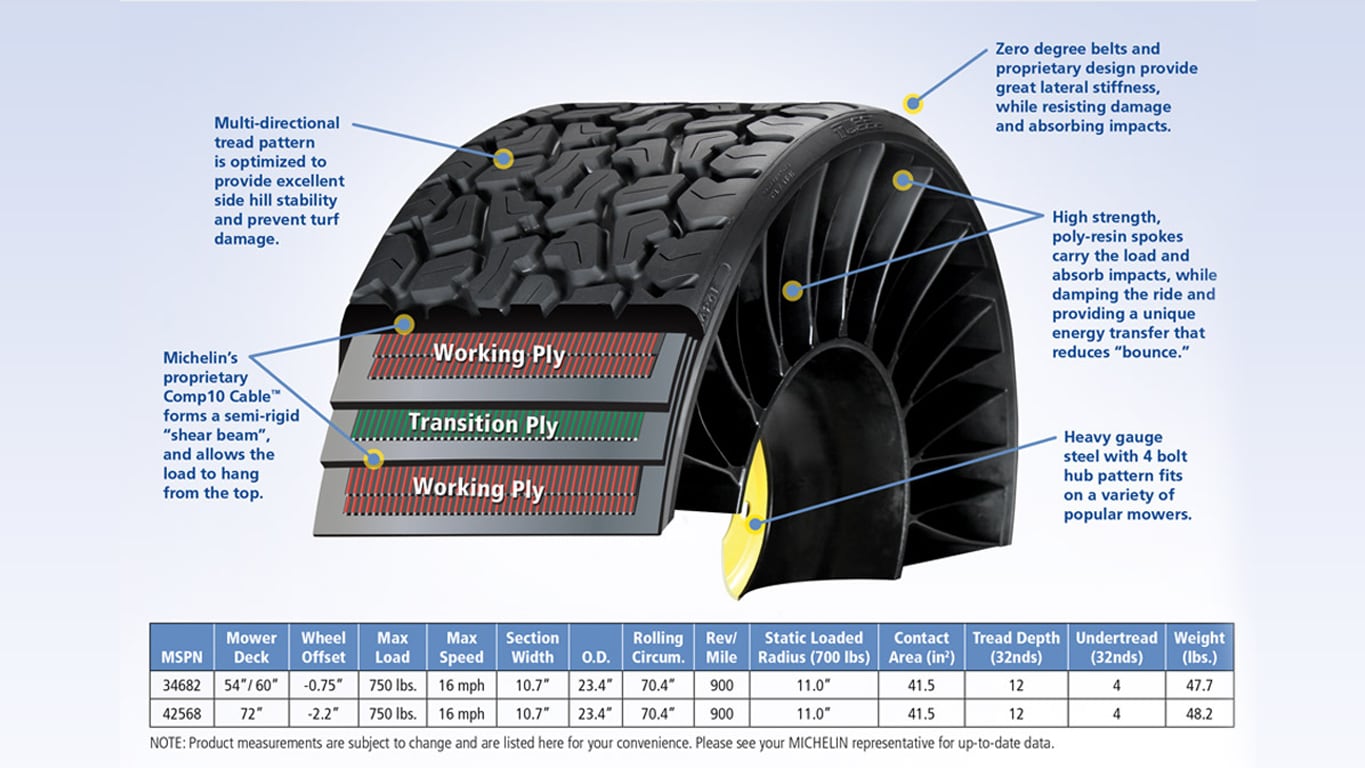This infographic features a detailed cross-section of a Michelin tire, set against a light blue, cloudy background. The tire is displayed in a horizontal landscape orientation and is meticulously labeled with various technical annotations and arrows pointing to different parts of the tire. The tire exhibits an aggressive off-road tread pattern, black in color, optimized for excellent side hill stability and turf damage prevention.

The cross-section reveals the tire's multi-layered structure, consisting of a red working ply, a green transition ply, and another red working ply. The tire components include high-strength polyresin spokes designed to carry the load, absorb impacts, and reduce bounce, thanks to the Polyresin's proprietary Comp 10 cable forming a semi-rigid shear beam. Zero-degree belts and a proprietary design provide significant lateral stiffness while resisting damage and absorbing impacts.

Further details highlight the tire’s construction, indicating that high-gauge steel with a four-belt hub pattern allows for compatibility with various mowers and industrial equipment. A table at the bottom of the infographic provides additional data, including maximum speed (14-16 miles per hour), maximum load, and other specifications in a two-row, 10-12 column format with a header row.

Overall, this infographic serves as a comprehensive guide to the tire's interior structure, durability, and suitability for specialized industrial applications, such as forklifts, warehouse equipment, or agricultural machinery.